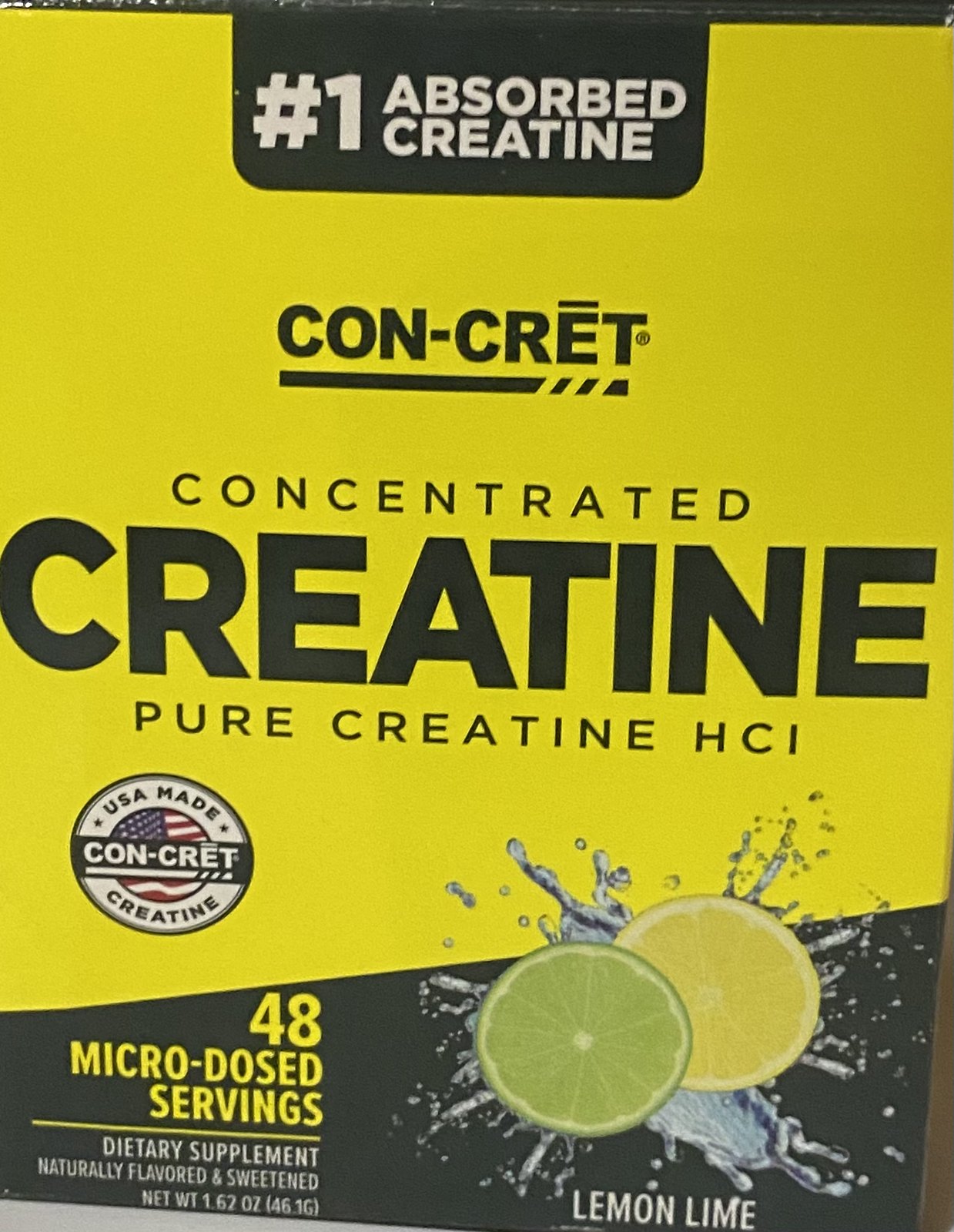This detailed up-close image showcases the packaging of a creatine supplement. The top two-thirds of the packaging is predominantly yellow with a prominent black rectangle at the top center. Within this rectangle, bold white text announces "#1 ABSORBED CREATINE". Below, the word "CON-CRET" appears in black with a horizontal line featuring breaks underlining "ET" and a registered trademark symbol. Beneath this, the text reads "CONCENTRATED CREATINE" and "PURE CREATINE HCI" in distinct black letters. 

On the yellow portion of the packaging, a black and white circle displays the text "USA MADE CON-CRET CREATINE," accompanied by a background featuring an American flag with red, white, and blue stripes and white stars. The lower quarter of the packaging shifts to a black background, highlighting vibrant imagery of a lemon and lime slice with splashes of water, enhancing the fresh theme. To the bottom left, in yellow text, it states "48 MICRO-DOSED SERVINGS." Below this, additional white text provides more product details. The right side notes that the product offers lemon-lime flavor.